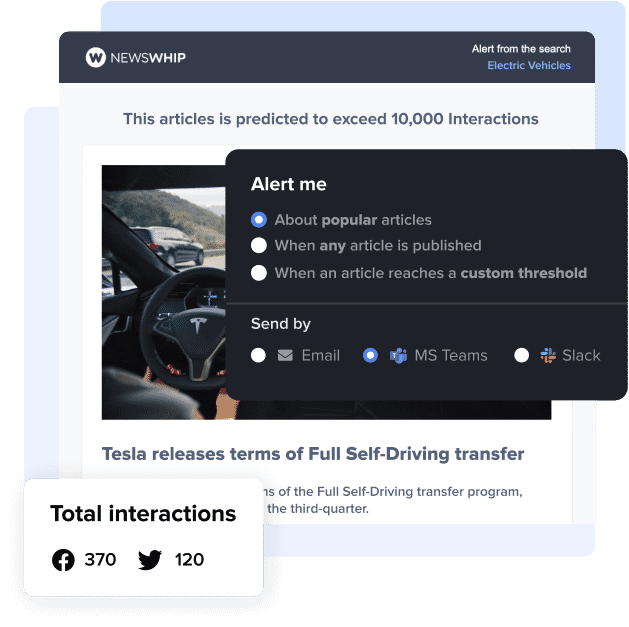On the News Whip website, a prominent black 'W' logo is encased in a white circle in the top left-hand corner, followed by the text "News Whip." This logo represents the company's brand. Adjacent to the logo on the top-line rectangular menu is an alert message indicating a search result for "Electric Vehicles." This message notifies the user of a relevant article, suggesting a previous search for electric vehicles on the platform.

The alert box reveals that this article is trending, with a prediction to exceed 10,000 interactions. Displayed below the alert is an interior image of a Tesla, enhancing the visual appeal of the notification. The alert box includes the cumulative interaction count, offering real-time engagement metrics. 

The highlighted article, titled "Tesla Releases Terms of Full Self-Driving Transfer," provides the latest update found by the search engine, aligning with the user's interest in electric vehicles.